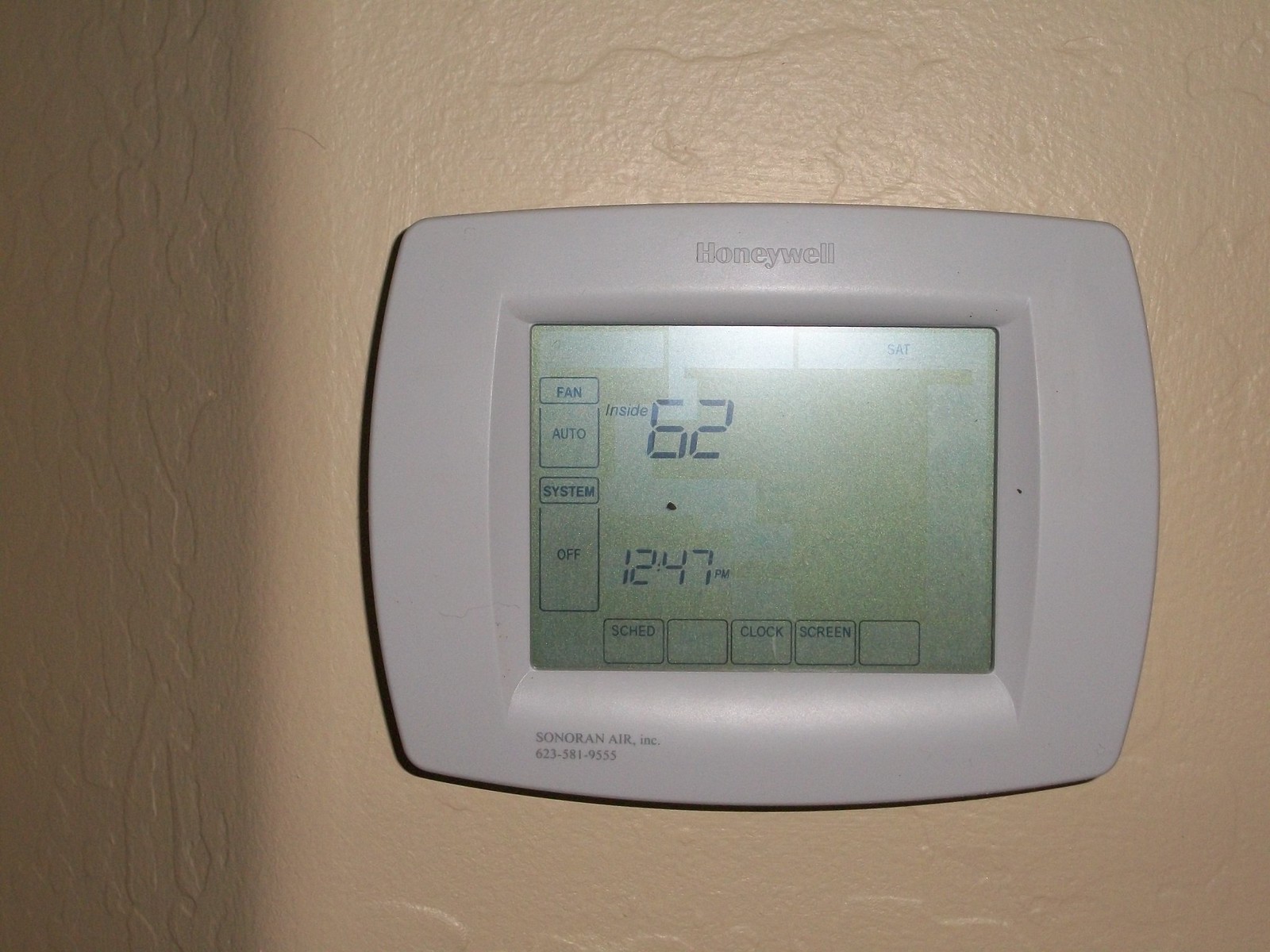Close-up of a digital thermostat, featuring a pristine white frame with the Honeywell brand name prominently displayed at the top. The bottom left corner of the frame bears the label "Sonoran Air, Inc." with a contact number, 623-581-9555. The thermostat's screen emits a green hue, displaying the current inside temperature at 62°F. On the left side of the screen, settings labeled "Fan" with the option "Auto," and "System" with the "Off" status, are encased in separate squares. The display also shows the current time at 12:47 PM. The lower section of the screen contains five squares, with the central one labeled "Sketch," flanked by an empty square on each side. Further to the right, two more squares are labeled "Clock" and "Screen," followed by another empty square.